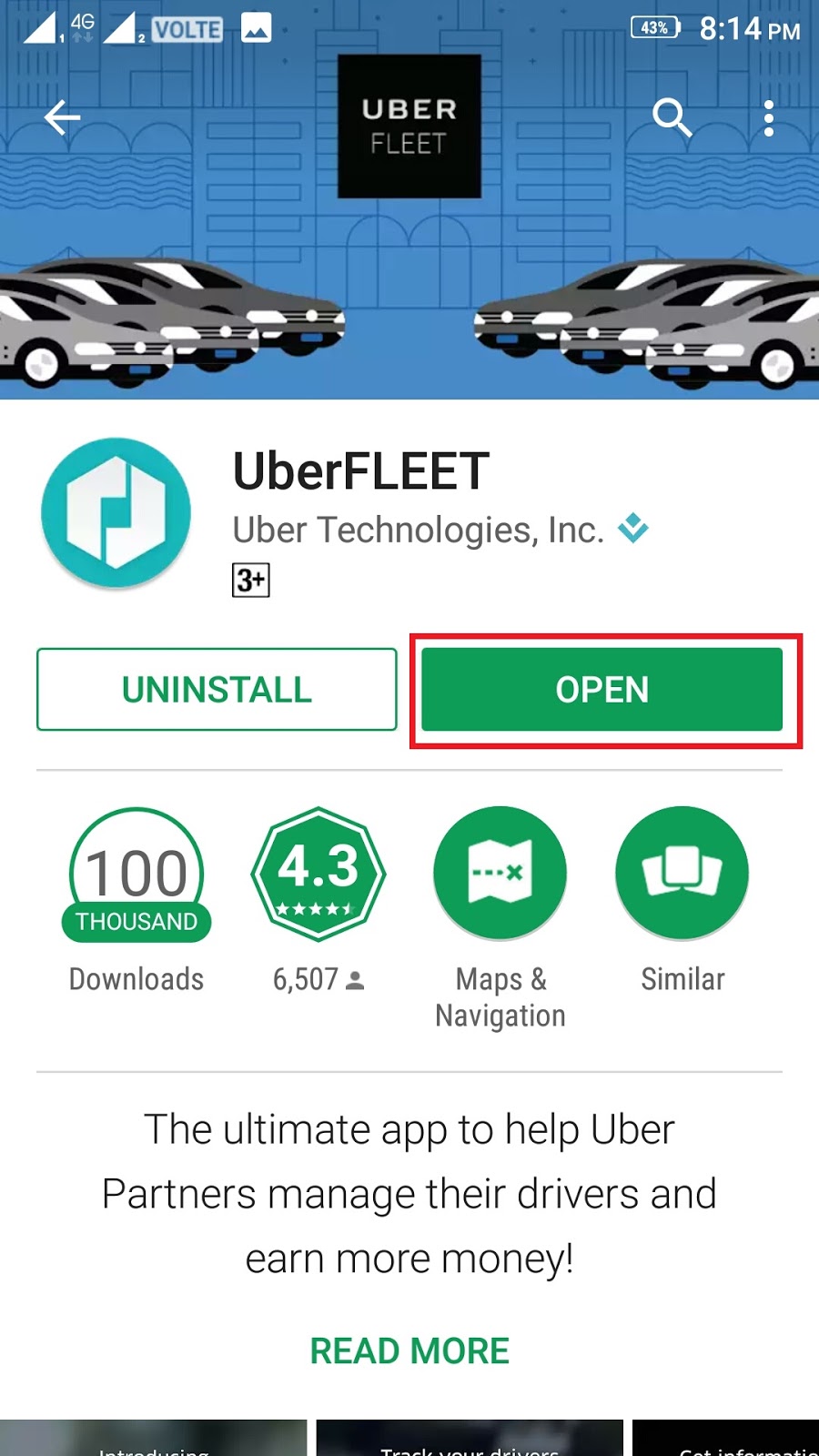The image displays a smartphone screen showing the Uber Fleet webpage. In the top left corner of the screen, "4G" indicates the phone's connectivity, while the battery icon on the right side shows that it is at 43% and the time reads 8:14 p.m. The webpage prominently features Uber Fleet at the top, with stylized illustrations of cars that have a cartoon or anime aesthetic. Below this, the words "Uber Fleet" and "Uber Technologies" are displayed alongside the Uber logo. 

Further down, there are two buttons: "Uninstall" and "Open," with the "Open" button highlighted in red. This option is likely emphasized for user convenience. The webpage mentions that the app has 1,000 downloads and is categorized under maps and navigation. It describes Uber Fleet as "the ultimate app to help Uber partners manage their drivers and earn more money." The image suggests that this individual is using the Uber Fleet application, catering to those who manage drivers for Uber.